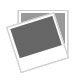The image displays two tags attached to a pair of beige, khaki-colored pants. The primary focus is on a tall, rectangular black-bordered tag with a white sticker in the center, affixed to the garment with a small plastic fastener. This black tag reads "Style: Matte Finish Khaki Twill" towards the top, followed by a code "M0033717009." Below the code, there is a barcode, and beneath the barcode, the tag indicates the composition of the fabric as "97% cotton, 3% elastane." It also features the size "31/30" and a recycling logo at the bottom right. Behind the black-bordered tag, there is a green tag that also contains a barcode. The background of the image is white, and the clothing item appears to be either shorts or pants, though the image is cut off, making it difficult to determine definitively.